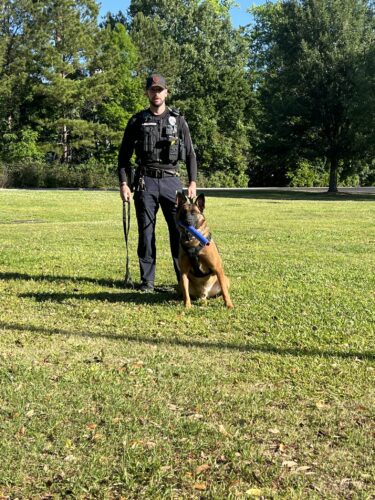The image features a police officer standing with a German Shepherd in a mowed, grassy field on a clear, sunny day. The background showcases a bright blue sky and an abundance of tall, green trees, creating a lush, verdant setting. The officer, a Caucasian male with a black beard and mustache, is centered in the photo and dressed in a complete black uniform, including a long-sleeve shirt, black pants, and a black baseball cap. His shirt, which doubles as a bulletproof vest, is adorned with various items such as a name tag, a shield, and other police equipment. He holds a black leash in his left hand, which leads to the German Shepherd sitting to his right. The dog, dark brown with black markings around its nose and ears, has a blue cylindrical toy in its mouth. The overall composition and detail suggest that this might be an official photograph for a police canine unit.